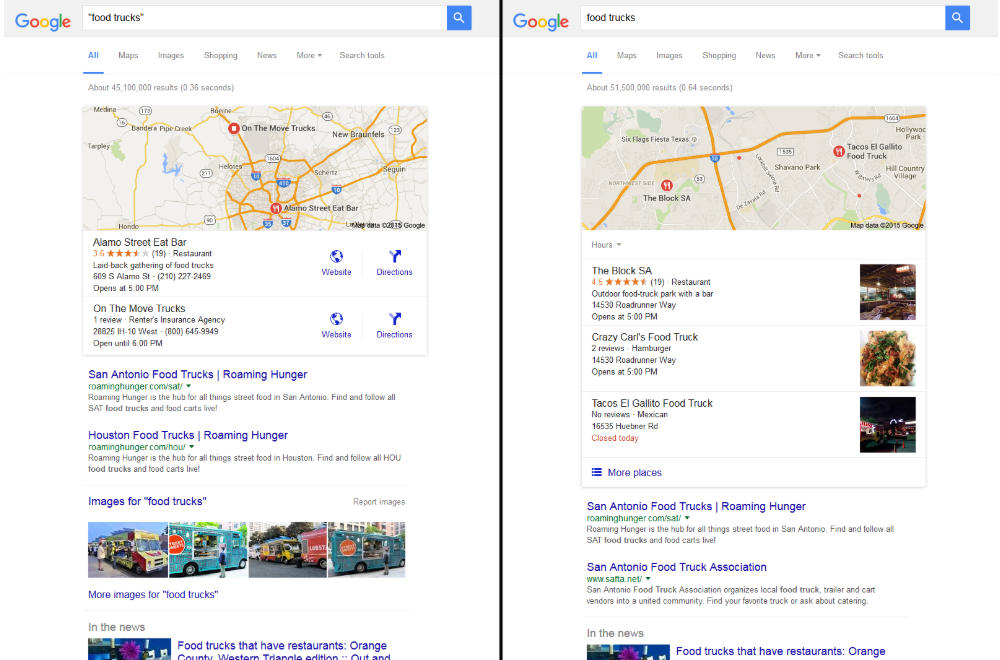This screenshot features two distinct Google search results displayed side by side. Both searches are for "food trucks," but the one on the left includes quotation marks ("food trucks"), while the search on the right does not. 

- **Left Search ("food trucks"):**
  - Results: 45,100,000 results
  - Top results include:
    - Alamo Street Eat Bar
    - On The Move Trucks
    - San Antonio Food Trucks (Roaming Hunger)

- **Right Search (food trucks without quotations):**
  - Results: 51,509,000 results
  - Top results include:
    - The Block S.A.
    - Crazy Carl's Food Truck
    - Tacos El Galito Food Truck

The screenshot illustrates the impact of using quotation marks in search queries on Google, yielding different results in both quantity and content.